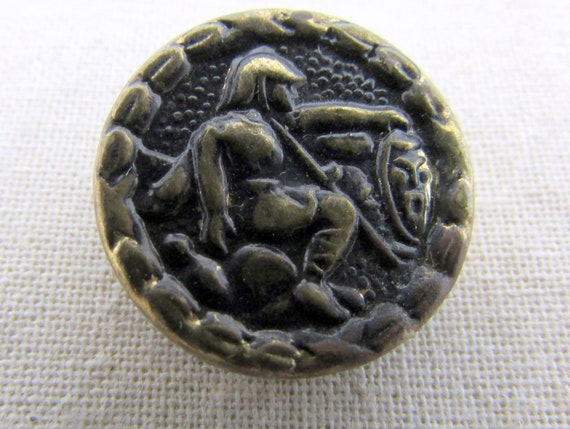The image shows an ancient, weathered coin or button with a bumpy, almost knotted edge resembling snake skin. The coin's metal appears to be a mix of black, brown, and golden hues, potentially suggesting a composition of copper and bronze with signs of aging, giving it a light bronze color with a greenish tint. The detailed illustration on the coin depicts a seated warrior or gladiator, viewed from the side. The warrior is wearing a helmet that extends to the back of his head. His right arm is stretched down with his hand outstretched, while his left hand appears to be holding a spear or staff. Near the warrior, there's a mask facing forward, showing detailed eyes, brows, nose, and a mouth. The coin rests on a fabric surface, adding to the impression of an ancient artifact.